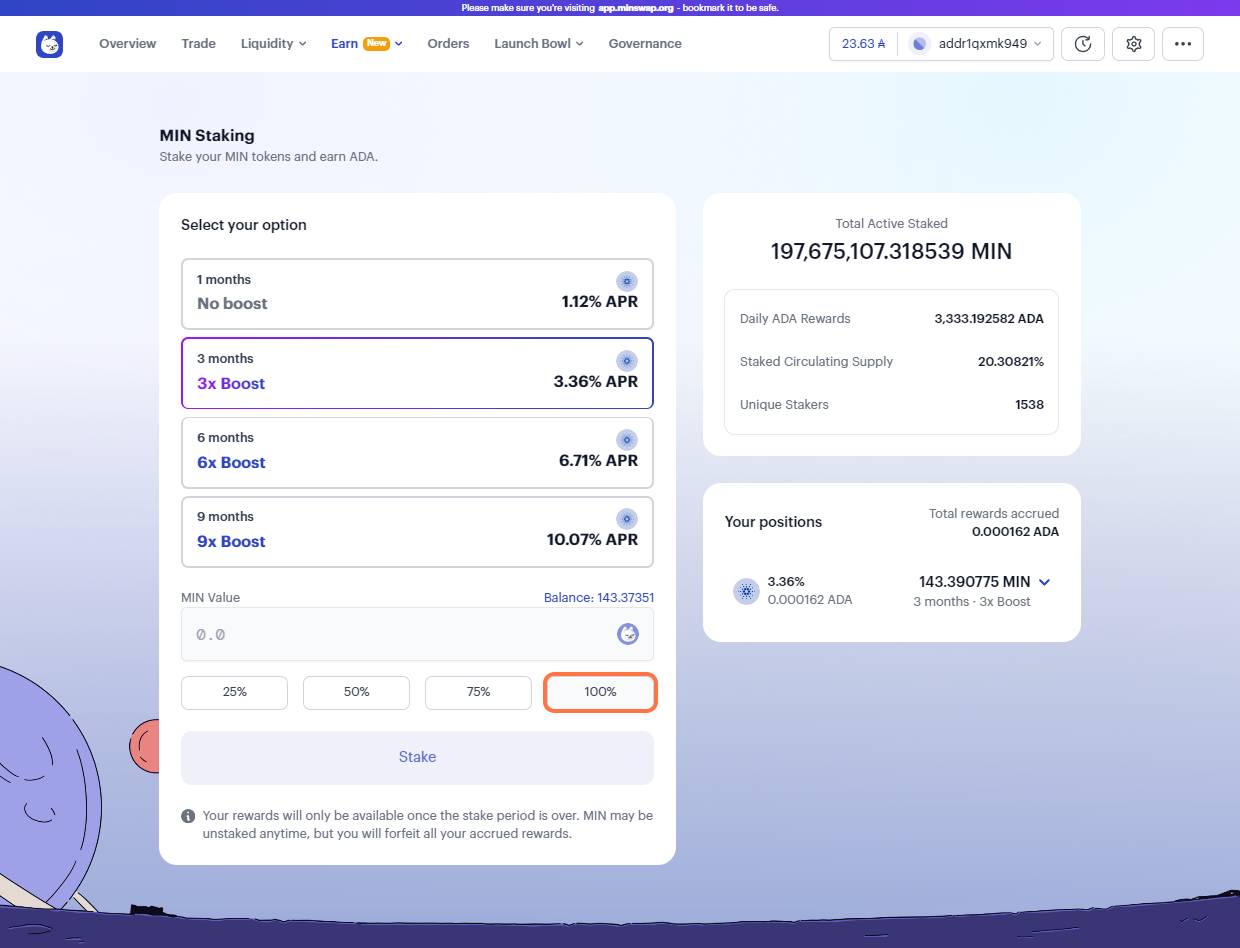This image is a screenshot of a web page interface for M.I.N. Staking. 

At the very top of the image, there is a narrow purple border with white text at the center, which is unfortunately too small to be legible. Directly below this is a white top menu bar. The company logo appears in the upper left of this menu, consisting of a purple square with rounded corners and a small, unidentifiable illustration within it. The company name, "M.I.N. Staking," is also displayed nearby in capital letters.

Moving from left to right, the top menu includes several items: Overview, Trade, Liquidity, Earn, Orders, Launch, and Governance. Beneath the menu, the background starts as a very light blue at the top, gradually transitioning to a bluish-purple hue towards the bottom.

In the center of the page, a prominent white rectangle contains key information. The headline "M.I.N. Staking" is at the top, followed by the subheading "Stake your M.I.N. tokens and earn ADA." Below this, the form for staking options is displayed. Four staking options are presented in a series of left-aligned rectangles:

1. One month - No boost
2. Three months - 3x boost
3. Six months - 6x boost
4. Nine months - 9x boost

Each option is paired with its respective Annual Percentage Rate (APR) on the right side. The one-month no boost option offers an APR of 1.12%. In contrast, the nine-month 9x boost option offers the highest APR of 10.07%.

To the right of these options, another rectangle is displayed with a smaller rectangle beneath it, although the exact purpose or content of these rectangles is not detailed.